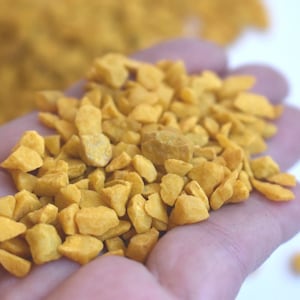The image depicts a person's hand held out flat, appearing somewhat light purple due to the lighting. The hand is filled with numerous small, rock-like items in various shapes and sizes, covering the palm and nearly reaching the fingertips. These items are predominantly yellow, with hues ranging from bright yellow to a darker shade, resembling a tannish camel color. Despite the blurriness of the image, it is evident that the yellow items are irregularly shaped, akin to cereal or possibly even dog food. In the background, there is a blurred area that suggests a larger pile of these yellow items, with a hint of light blue that might be a table or the surface from which they were picked. The items in the hand are piled high, with some on the verge of falling off the edges.